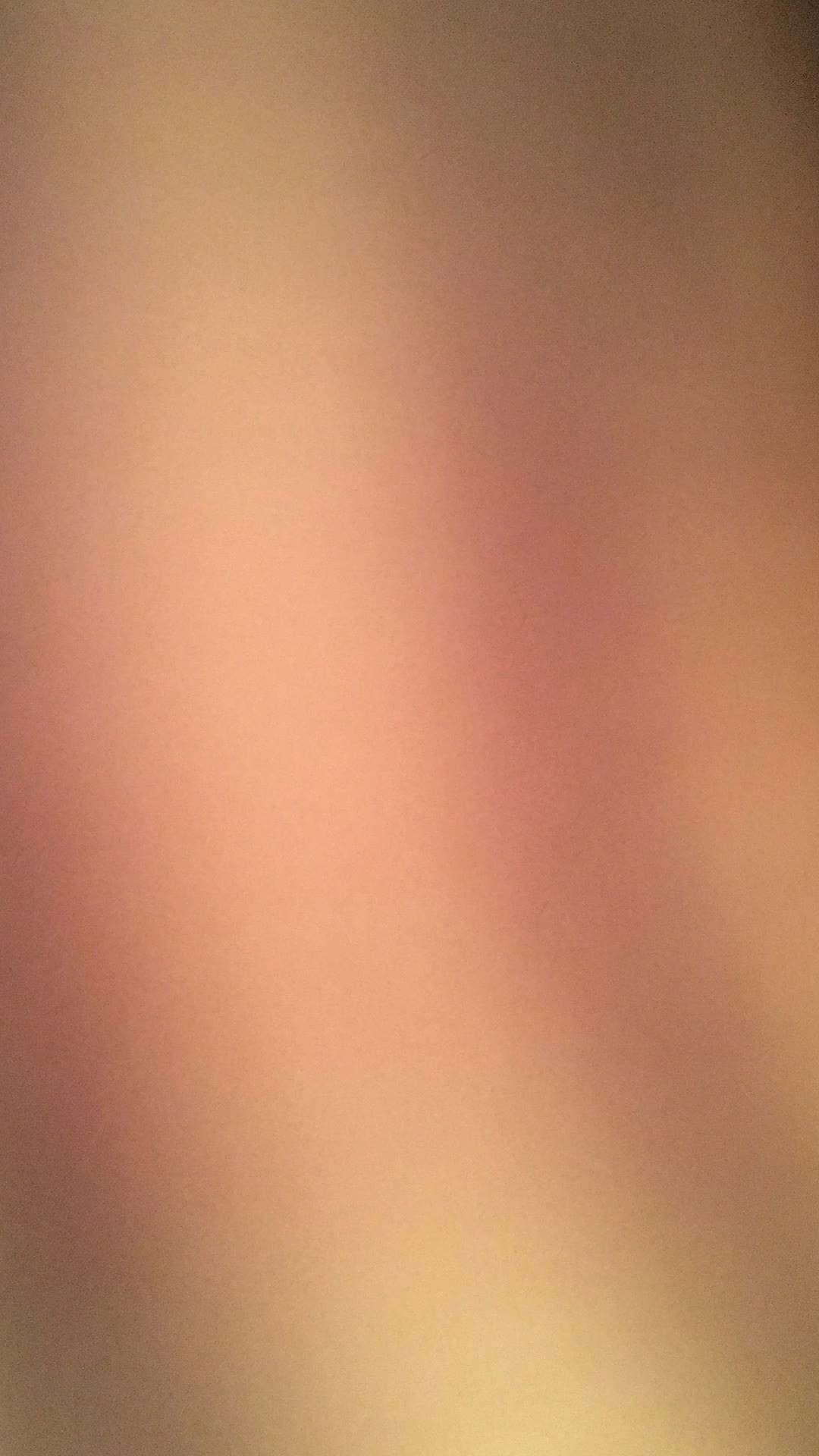A detailed close-up image of a textured surface prominently featuring colors and tones reminiscent of human skin. The central area includes subtle yellowish and pink hues, alongside distinct red streaks running vertically. The overall appearance suggests the pigmentation of a light-skinned individual, although the flawless nature of the surface implies it may be artificially created or digitally rendered, possibly simulating skin or covered in makeup for a uniform look. The image captures the intricate interplay of colors and textures, evoking the impression of an extremely smooth, unblemished dermatological sample.